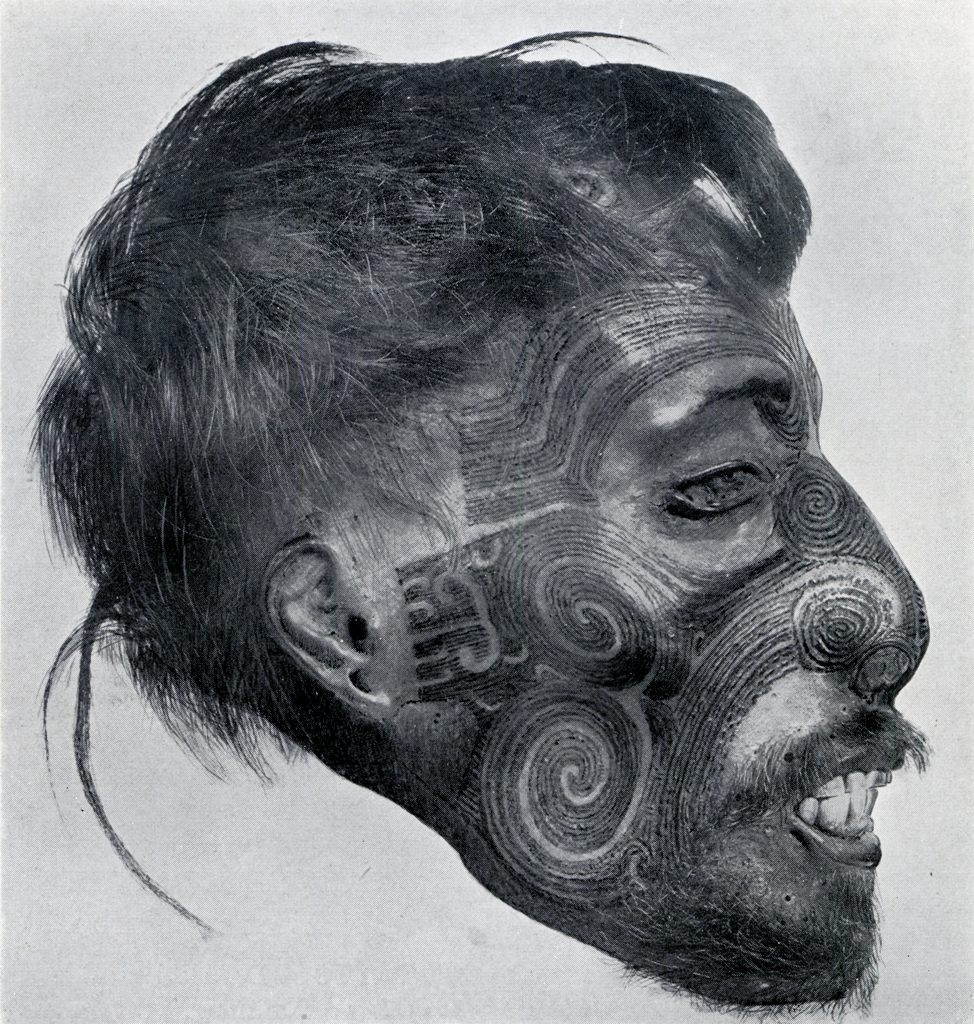The image portrays a detailed side profile of a man's head, adorned extensively with tattoos that cover most of his face in intricate, swirling patterns. His hair is predominantly black but appears messy and matted, with a single long piece of hair trailing down to the left and some shorter strands hanging halfway down his forehead. Notably, the man's nose is long and ridged, with design elements curving up and around it in clockwise and counterclockwise directions. His eyes seem sealed shut, creating an almost lifeless appearance. The mouth is open, revealing top and bottom teeth, which are notably square. A thin beard and mustache frame his mouth, and his thin earlobe is pierced with a large hole. The ear uniquely features a black dot and multiple holes. The background of the image is a grayish-white, enhancing the predominantly black-and-white contrast of the tattooed face, giving it a somewhat archaic, caveman-like, or even monkey-like visage.